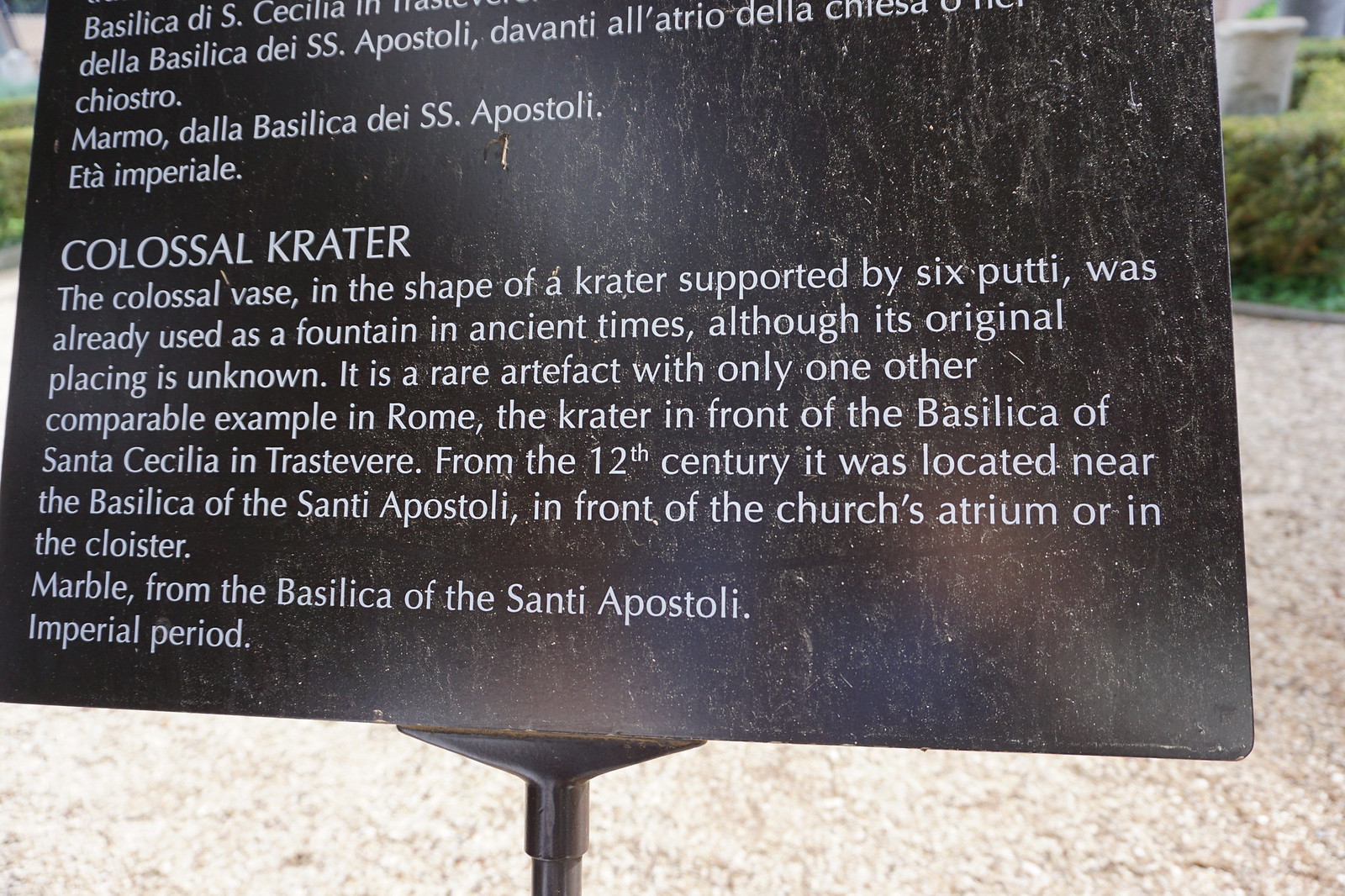The image showcases a wide rectangular outdoor sign on a black metal slab that appears dirty, adorned with tiny grayish white specks and scratches. The black pole supporting the sign is slightly to the left of the center at the bottom of the image and is also cut off. Below, light gray cobblestones are visible, and green bushes form the backdrop. The top portion of the sign, written in Italian, is cut off, but the visible part in white font reads: "Colossal Crater: The colossal vase in the shape of a crater, supported by six putti, was already used as a fountain in ancient times, although its original placing is unknown." The paragraph continues, discussing its historical significance and rare nature, noting another similar artifact in Rome and its connections to the Basilica of Santa Cecilia in Travestere and the Basilica of the Santae Apostoli. The information suggests that the sign is placed outdoors, possibly on a sidewalk, accentuated by the surrounding natural elements.